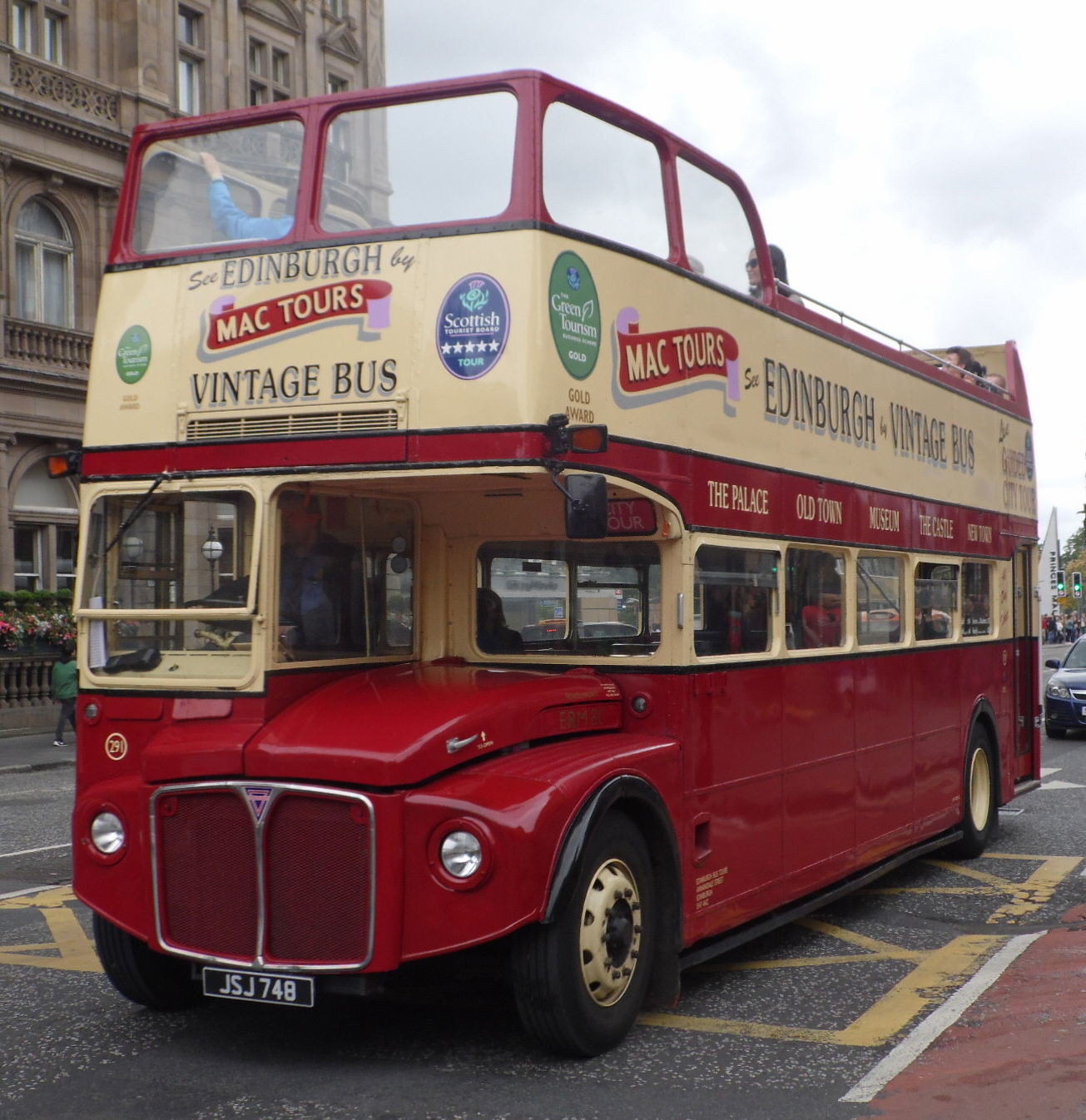The image is a large square photograph featuring a classic double-decker bus parked in the parking lane on a road. The bus is predominantly red on the bottom with an open top upstairs, bordered by a tan or beige color. Prominent text on the side reads "Edinburgh Vintage Bus Mac Tours," and there are labels indicating a "Scottish Tour" with five stars beneath it, along with another label for "Green Tourism." The bus has a visible conductor at the steering wheel on the right side and a license plate reading "JSJ 748" in white letters on a black background. There are a few passengers visible on both the open-top upper deck and the enclosed lower level. The road it’s parked on appears worn, and across the street in the upper left of the image, a multi-story brownstone building with arched windows is evident, contributing to a European, urban ambiance. The sky in the upper right corner is filled with a blend of gray and white clouds, suggesting overcast weather.